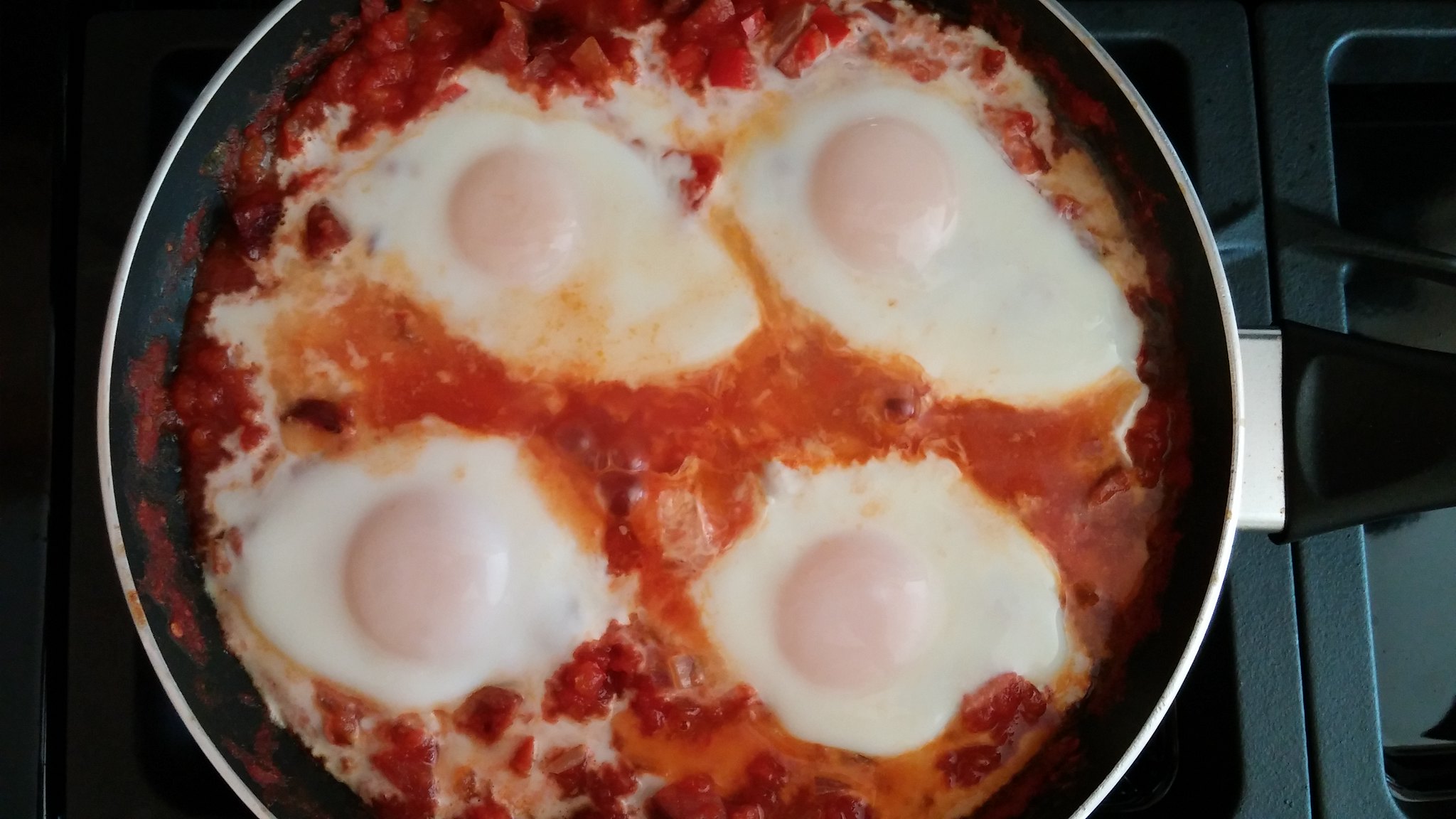In this overhead shot, a black, Teflon-coated metal frying pan with a black handle sits on a clean gas stove with a black frame. Inside the pan, four eggs are cooking, their yolks prominently standing out against the surrounding egg whites. Interspersed among the eggs are bits and pieces of bacon and a vibrant red tomato sauce, creating a visually striking contrast. The pan's position reveals two gas burners partially in view. The overall composition highlights the meticulous preparation of a savory dish, likely a variation of eggs poached in a tomato-bacon mixture.